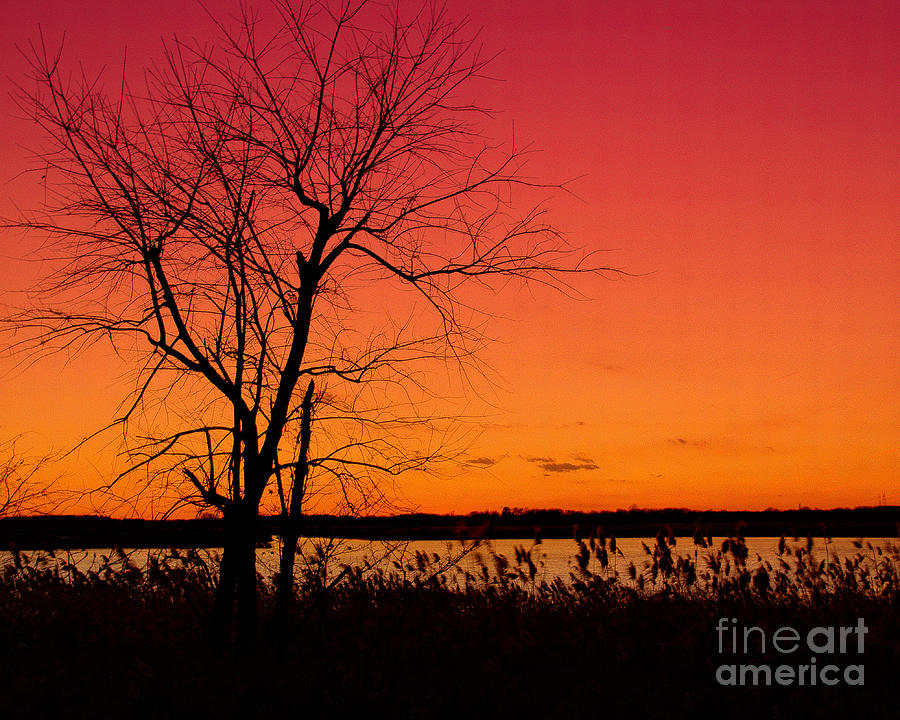An artistic photograph captures a breathtaking wintertime sunset, featuring a dramatic gradient in the sky—from deep, rich red at the top to vibrant orange near the horizon. Centered in the foreground, a tall, leafless tree with multiple branches stands as a stark silhouette against the radiant backdrop. The intricate web of branches allows the mesmerizing shades of red and orange to peek through, adding depth and warmth to the scene. Below the tree, the water, possibly a river or lake, beautifully mirrors the glowing colors of the sky, enhancing the overall brilliance. Silhouetted silhouettes of smaller plants and tall grass, typical of those found along a shoreline, are visible at the bottom, adding a delicate texture to the composition. The image carries the watermark “Fine Art America” at the bottom right, subtly marking its artistic origin.